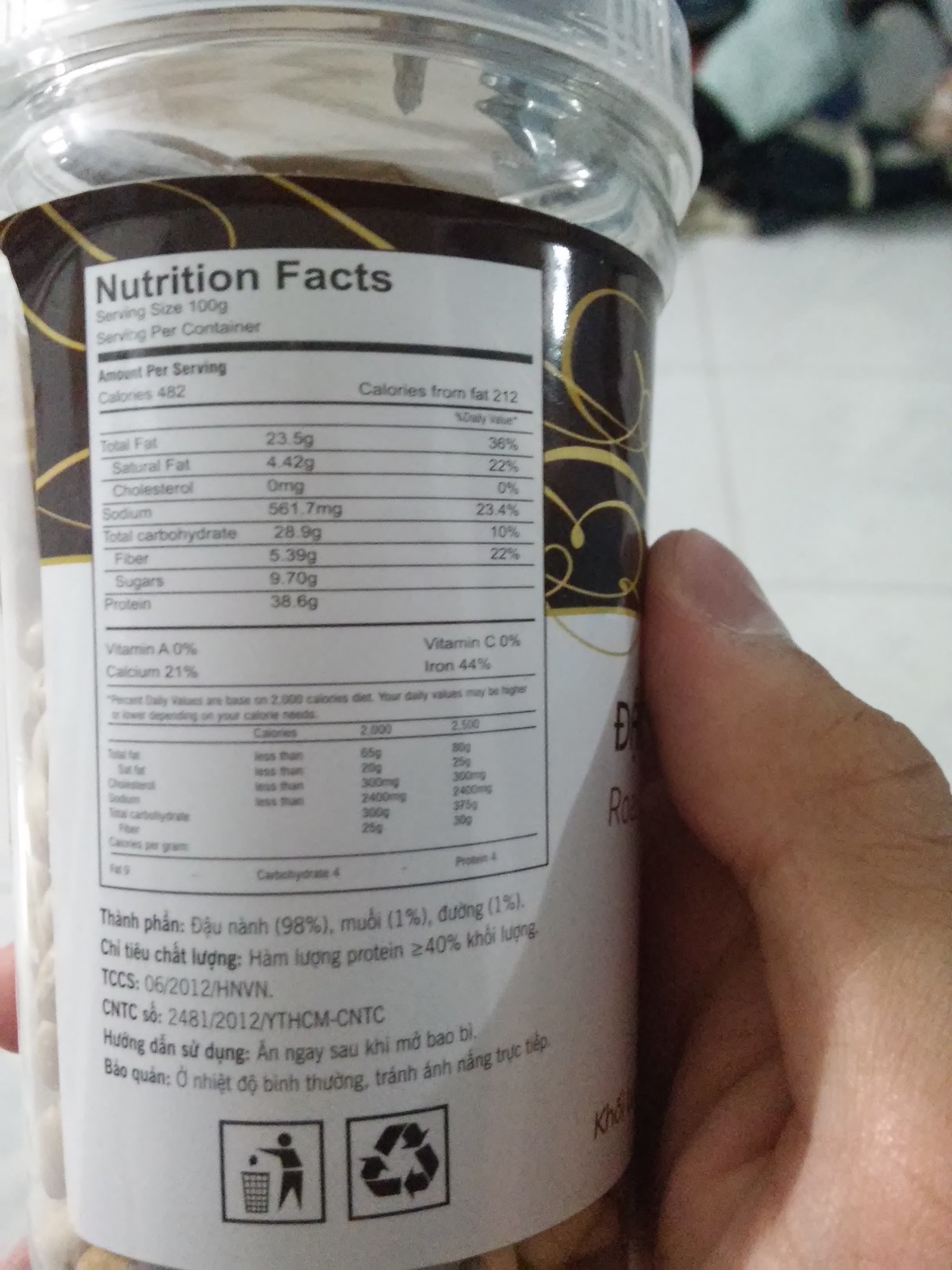In this portrait-style photograph, a light-skinned individual holds a jar or bottle of food with the nutrition facts prominently facing the camera. The bottle is carefully rotated to display the nutrition label, obscuring the product's identity. The person's thumb is visibly gripping the jar. According to the label, a serving size is 100 grams. It lists 482 calories per serving, with 212 calories originating from fat. The product contains 23.5 grams of fat, 561.7 milligrams of sodium, and 28.9 grams of total carbohydrates. Of the total carbs, 5.39 grams are from dietary fiber, and 9.7 grams are sugars. The number of servings per container is not specified.